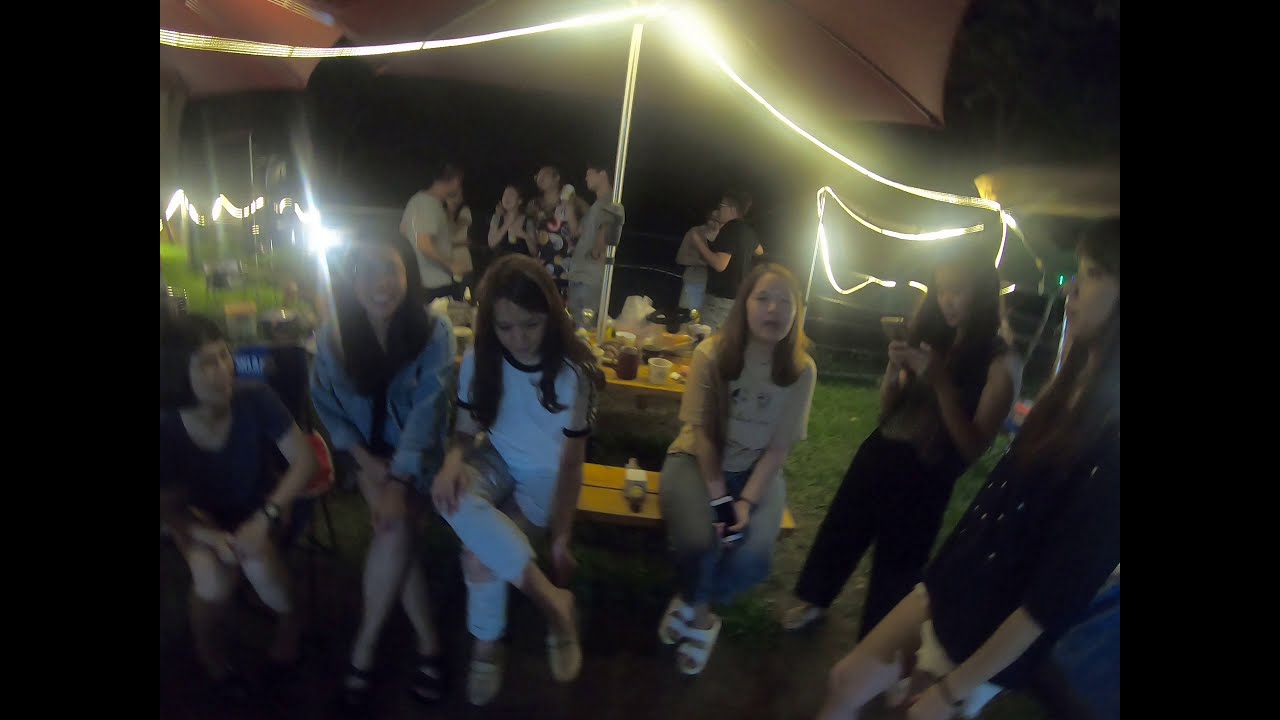In this nighttime outdoor party scene, possibly in a city or backyard, the dark sky is illuminated by bright string lights hanging overhead and causing some glare in the photograph. The scene is set around green grass with picnic tables and folding camp chairs scattered around. The overhanging structures, possibly reddish or orangish patio umbrellas, are supported by poles. In the mid-ground, four young women are seated at a yellow picnic table that is full of various foodstuffs, with one woman crouching beside them. Another woman stands next to the table, and one more is in the foreground, looking off to the left. To the right, closest to the viewer, are six women dressed in a mix of casual attire—black shirts, green pants, tan tops with jeans, a denim jacket, and black short-sleeved shirts, all wearing sandals. In the background, a group of men and women engage in conversation, and a young couple stands a bit farther behind them. The entire scene is framed by the bright string lights that add a festive glow to the gathering.